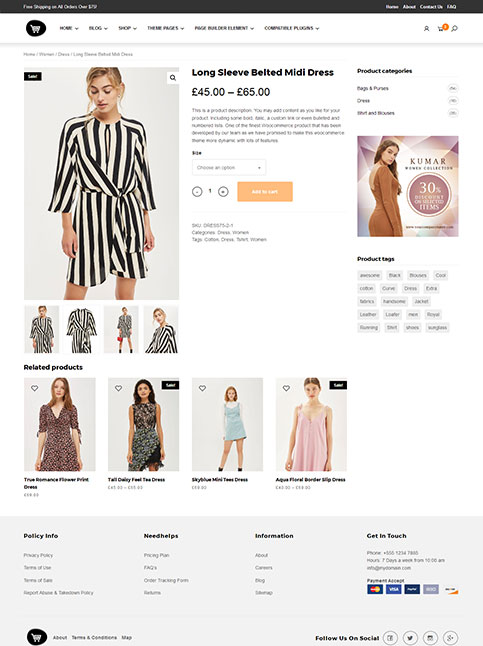In this image, we see a screenshot of a website with a black bar header at the top, featuring navigational links such as "About" and "Contact Us" on the upper right corner. On the left side of the header, there is a text that mentions "Free shipping on all orders over..." (the remainder is unreadable due to blurriness). Next to the text is an icon of a white shopping cart within a black circle.

Below the header is a large photo of a young, blonde model wearing a black and white striped, long-sleeve, belted midi dress. The dress is priced between 45 and 65 pounds. Directly under this description, an action button in bright orange reads "Add to cart," accompanied by a quantity selector featuring a minus and plus sign with the number one in between.

To the right of the main image, there is a small advertisement featuring another young woman wearing a brown dress, likely advertising a brand called "Kumar." Beneath this image, it says "30% off," and the word "items" is visible, indicating a discount on multiple products.